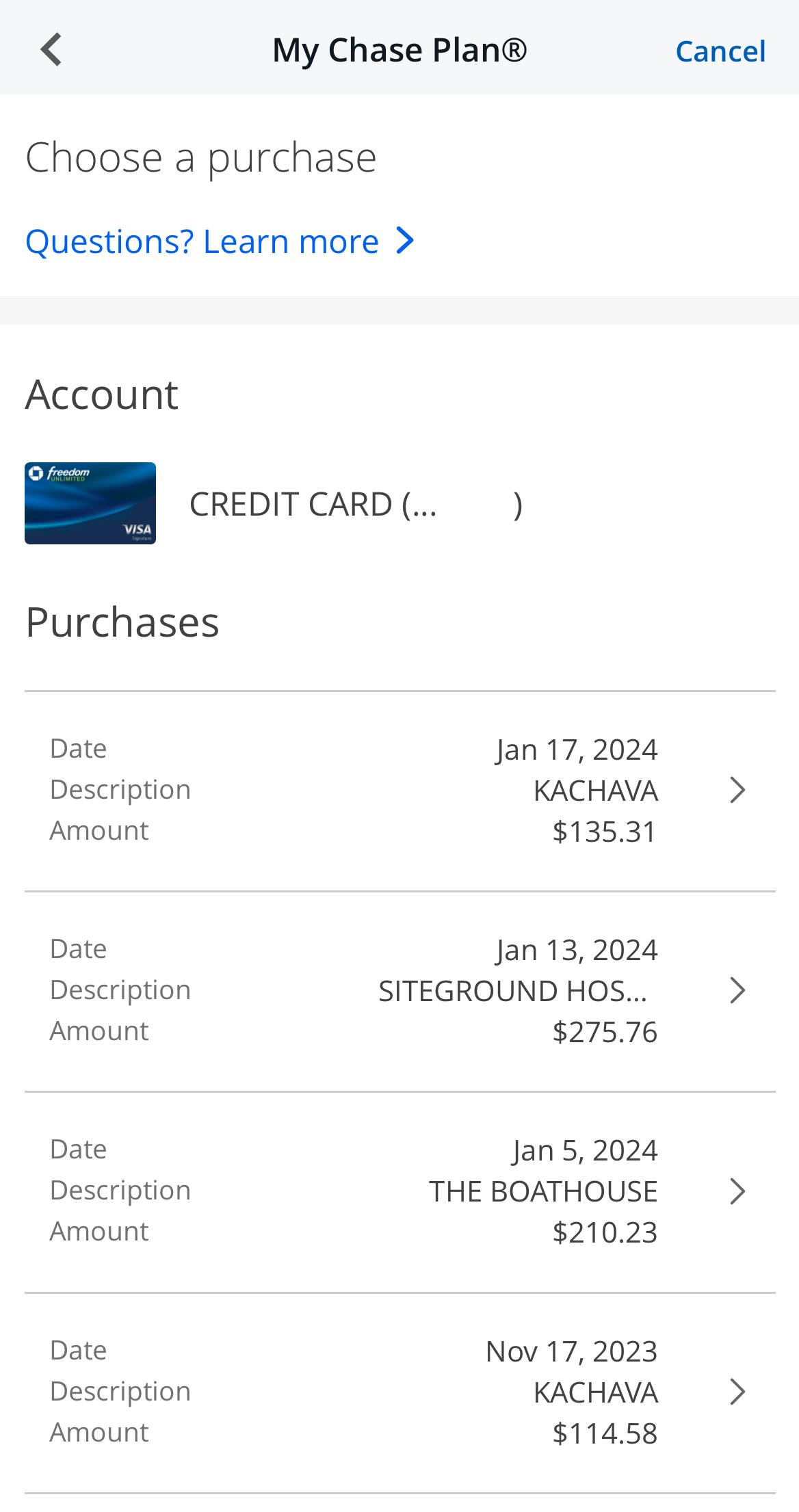The image displays a user interface for a financial tool titled "My Chase Plan." At the top of the screen is a light gray box containing a left-pointing arrow and the text "My Chase Plan" in the center, with a blue hyperlink labeled "Cancel" on the right. Below this, on a white background, is the prompt "Choose a Purchase," accompanied by a blue hyperlink reading "Learn More," along with a right-pointing arrow.

A light gray horizontal line separates the top section from the content below. The next section starts with the header "Account," featuring an image of a blue credit card to the left and the label "CREDIT CARD" in capital letters on the right, enclosed by parentheses with three periods "(...)" inside.

Following another horizontal line, the section titled "Purchases" details individual transactions:

- The first entry, under the heading "Date," shows "January 17, 2024." Beneath "Description," it reads "Kachaba," while under "Amount," it lists "$135.31."
- Another transaction, beneath the "Date" header, shows "January 13, 2024." The "Description" denotes "SiteGround HOS," and the "Amount" is "$275.76."
- A third entry lists the "Date" as "January 5, 2024," though the "Description" and "Amount" fields are out of the frame.

Each transaction is separated by horizontal lines for clear delineation.